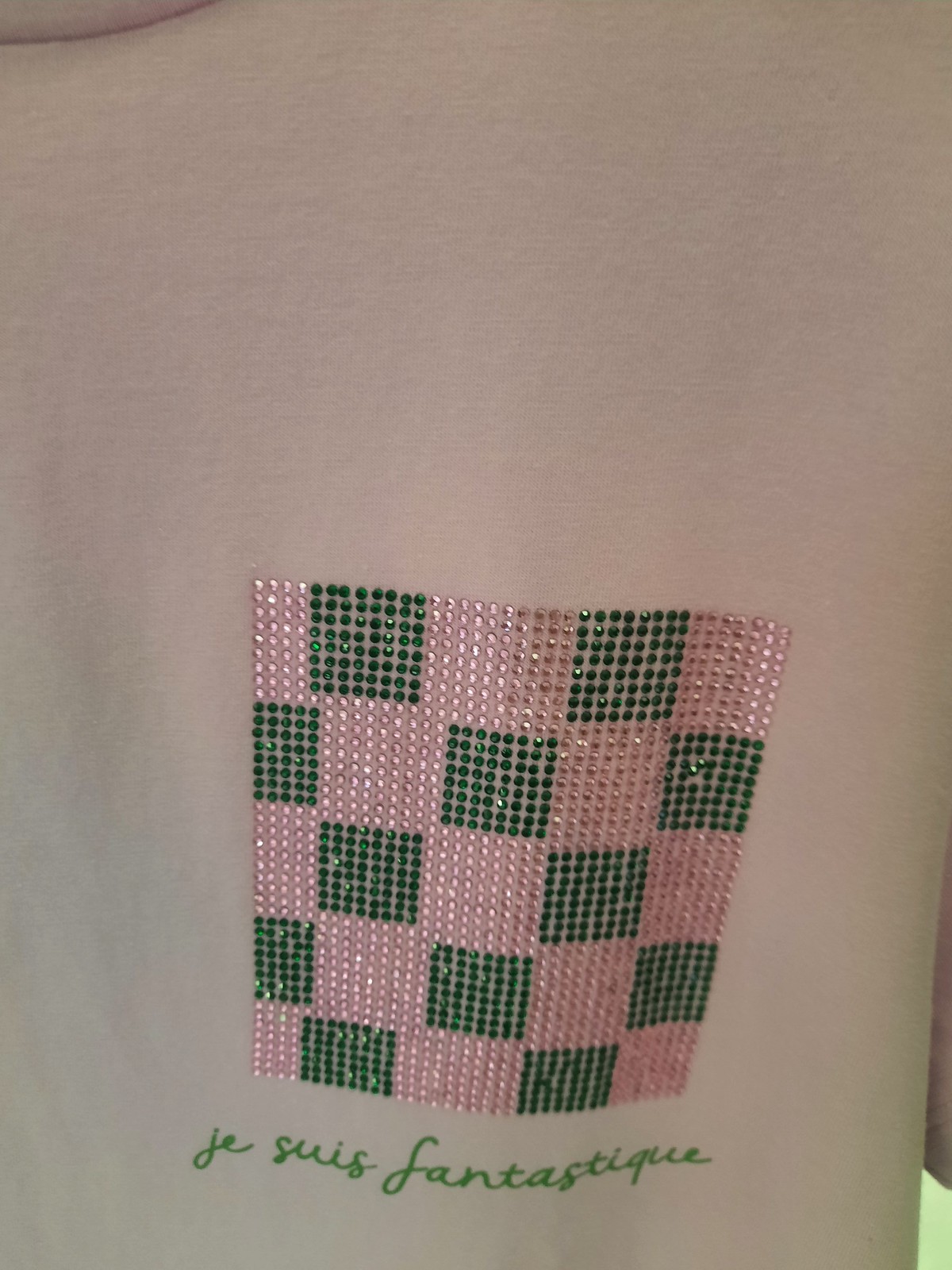The image displays a close-up of a white t-shirt being worn, with the photo so closely zoomed in that only a hint of the shirt's collar is visible in the top left corner. The upper third of the image is composed entirely of plain white fabric. Capturing attention in the lower third is an intricate decoration: a square checkerboard pattern made of small crystals or jewels. This decorative square is divided into a 5 by 5 grid, where each smaller square within the grid is filled with a meticulous 8 by 8 arrangement of tiny gemstones. The gemstones alternate between pale pink and forest green, creating a visually striking pattern. Below this jeweled design, elegant text in a lively spring green script reads, "Je suis fantastique."